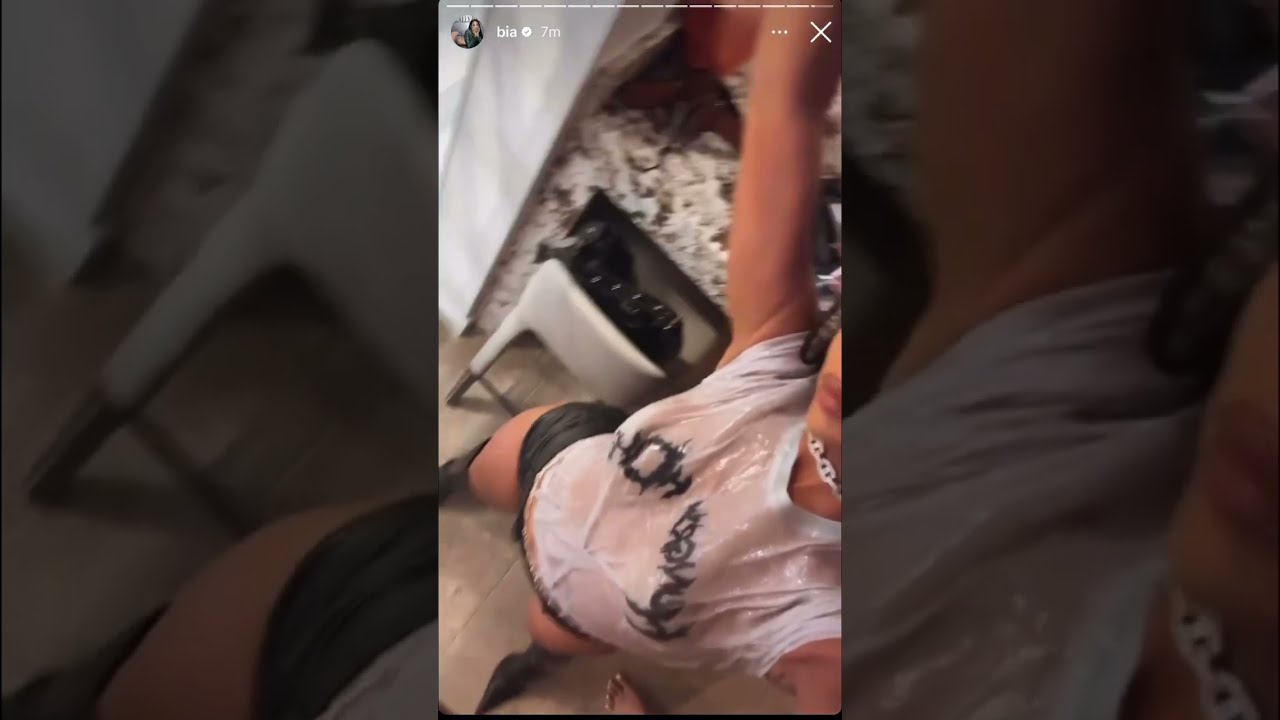The image is a vertical, smartphone-style photograph that seems to be part of an Instagram reel. The main picture is centrally placed, taken in a selfie-style with the camera angled downward at the woman's body. In the image, the woman has large, puffy lips coated in pink lipstick, which look like they might have had plastic surgery. She is wearing a tight, silver choker around her neck and a see-through, wet white shirt with indistinct black writing on it. Below, she dons very short, black leather-like shorts, complemented by tall black boots with pointy toes. 

The background of the photograph is the same image, but zoomed in and blurred, creating a faded border effect. The setting appears to be an interior environment with a stone floor. Behind the woman, there is a small off-white chair and what looks like a granite-color desk with a drawer. On the desk, there seems to be an orange object, though it is partially obscured. The Instagram interface elements are visible at the top of the image, indicating the reel was posted seven minutes ago by a user with the handle "BIA". The woman's complexion is a dark brown tone, and the overall composition highlights both the fashion elements she is wearing and the surrounding environment.